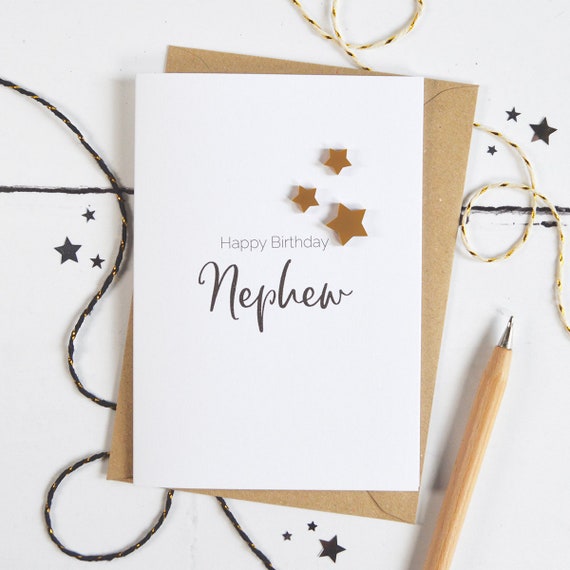This image features a neatly arranged birthday card setup. The white birthday card, with a simple design, reads "Happy Birthday Nephew" - "Happy Birthday" is displayed in gray letters and "Nephew" in larger, cursive brown letters. Surrounding the text are small brown stars: three placed to the right above the "Happy Birthday" greeting and others scattered on the left, center, and bottom of the card. The card sits atop a brown envelope, and alongside the envelope, a wooden pen with a silver tip rests to the right. Below the envelope is a background that hints at an underlying package, decorated with strings in two designs—one black with yellow specks and another sand-colored with yellow accents. Additionally, the overall background of the image is white with a faint black paint streak. The image's composition is thoughtfully laid out, emphasizing the birthday greeting occasion.